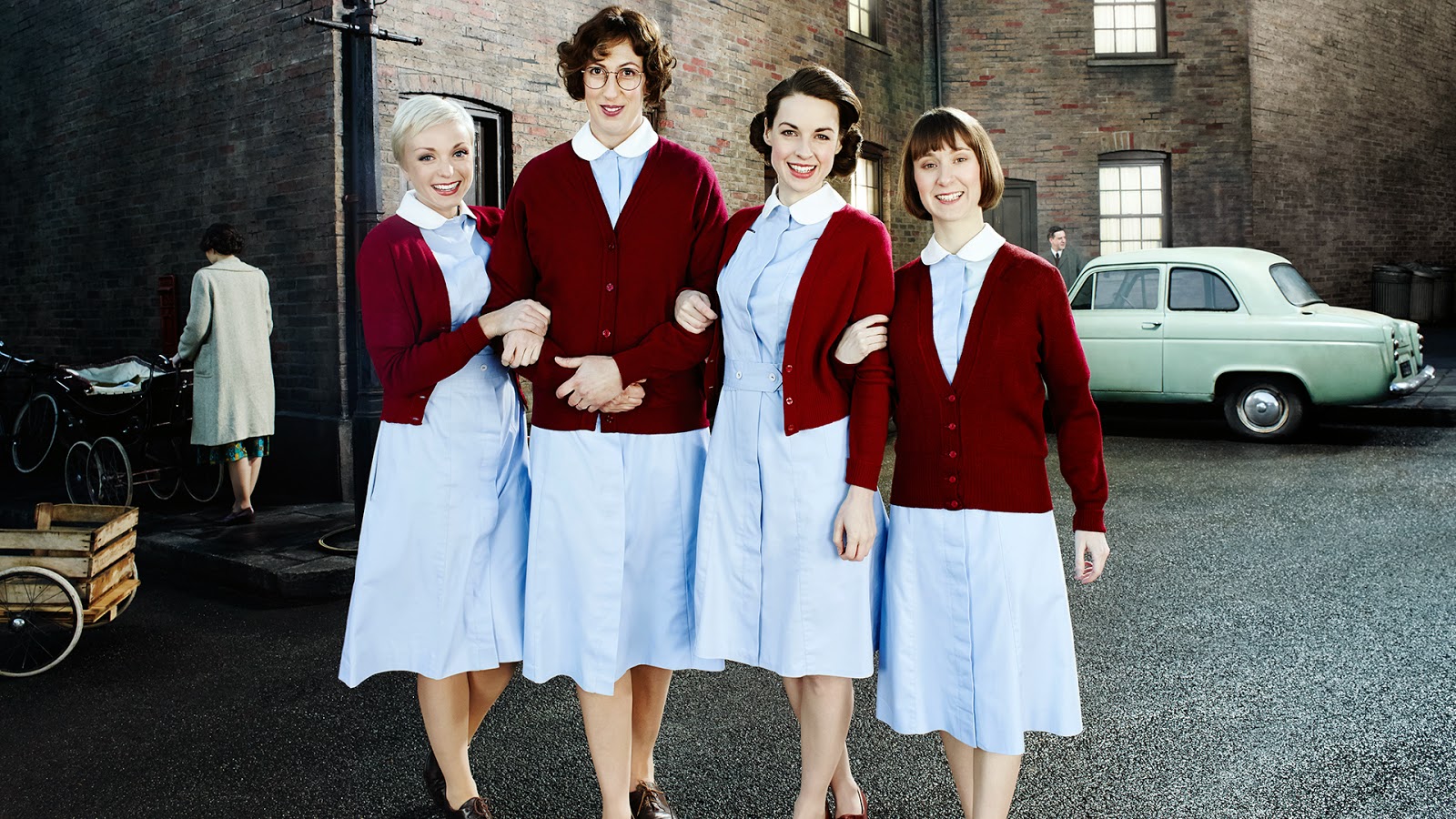This color photograph features four women posing outside on a dark gray gravel street, dressed in matching outfits that might suggest they are either students, perhaps members of a college sorority, or nurses from an earlier era. Each woman is wearing a light blue, knee-length dress with white lapels at the collar, paired with maroon V-neck cardigans and brown shoes. The women stand with their legs crossed and their arms linked, all smiling and wearing red lipstick. 

From left to right, the first woman has short blonde hair and is smiling. Next to her is a tall woman with short, curly reddish-brown hair and glasses. The third woman has her brunette hair pinned back, while the fourth has a lighter brown bob with bangs. 

In the background, to the left, there is a woman pushing a baby carriage, dressed in a long white coat, and to the right, a light green vintage two-door car, with a man standing nearby. They stand in front of a stone building with dark colors—black, brown, and dark red bricks—accenting the structure.